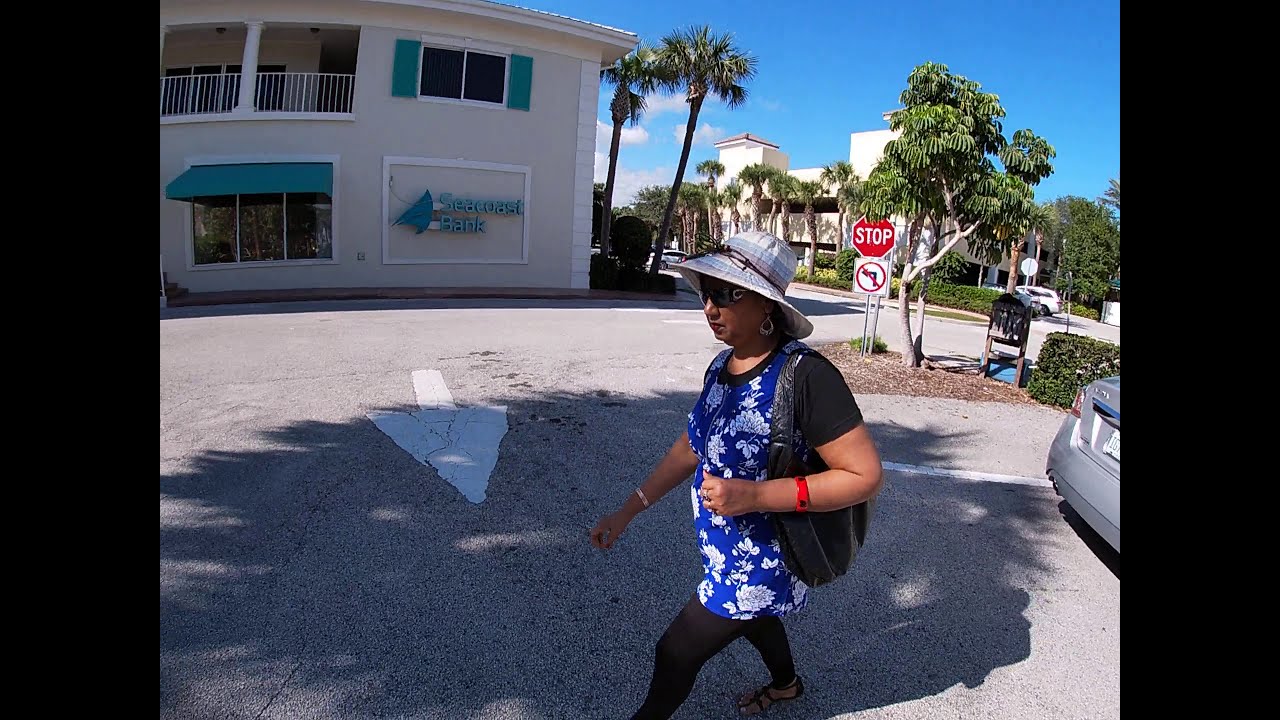The image depicts a sunlit and vibrant scene in what appears to be a tropical or beachside community. At the center, a woman with light brown skin is walking from right to left, captured in her left side profile. She is adorned in a blue top with a white floral pattern, paired with black capris and black leggings. She complements her outfit with a large, floppy gray hat and thick black sunglasses, adding a touch of elegance with silver hoop earrings. Carrying a black bag over her left shoulder, she has a distinct red bracelet on her left wrist and a white watch on her right.

The scene is set in a parking lot or along the side of a road, with a distinct fisheye effect that slightly distorts the view. A white directional arrow on the ground points towards the viewer, while a gray or silver car is parked behind her to the right. The background is rich with palm trees and clear blue skies, enhancing the sunny and inviting atmosphere. Across the street, several buildings are visible, including a small motel, a mid-century styled Seacoast Bank with teal shutters and an overhang, and a large white building that resembles a hospital or urgent care facility. The image is framed with a black border on the left and right sides, adding a finishing touch to the composition.